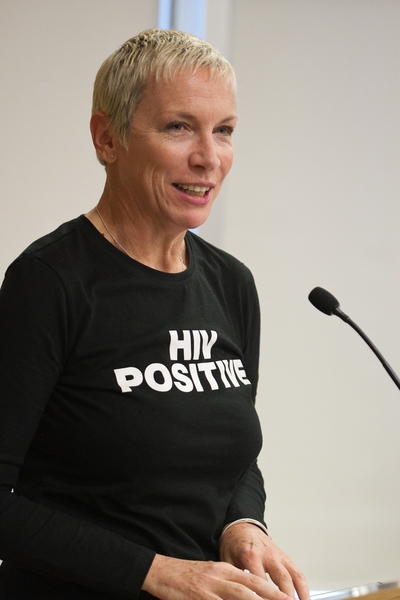The photograph captures a woman in her late 40s or early 50s, standing at a wooden podium. She has very short, bleached blonde hair and dark eyebrows. The woman is speaking into a black microphone that extends from the center-right of the image toward her face. She is wearing a long-sleeved black shirt with the bold, white capital letters "HIV POSITIVE" emblazoned across the chest. Her mouth is open, showing her teeth, suggesting she is either actively speaking or mid-smile. Her hands rest on the podium, and she wears stud earrings and two bracelets on her left wrist. The background is a bluish-gray, with an off-white wall featuring a window above her head, indicating she might be in a large hall or similar setting. The detailed image highlights the woman's focused and possibly empowering stance as she addresses her audience.